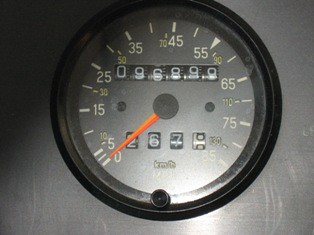This photograph features an analog car dashboard gauge highlighted by an orange needle that vividly displays the vehicle's speed in miles per hour and its engine revolutions per minute (RPM). The needle, bright orangish-yellow in color, stands out prominently against the black-rimmed gauge. A small adjustment button is located at the bottom, likely used for resetting the mileage or making other adjustments. The gauge needle currently points to zero, indicating that the car is stationary at the time of the photo. The mileage displayed is also analog, presenting a reading of 96,899 miles.

The gauge measures speeds up to 130 kilometers per hour and RPM up to approximately 85,000, suggesting that this is a European car adhering to the metric system. The dashboard is framed in stainless steel, contributing to a sleek and modern aesthetic. A bright glare is visible at the bottom of the image, suggesting that the photo was taken with a phone in low lighting conditions, causing the camera's flash or ambient reflections to appear.